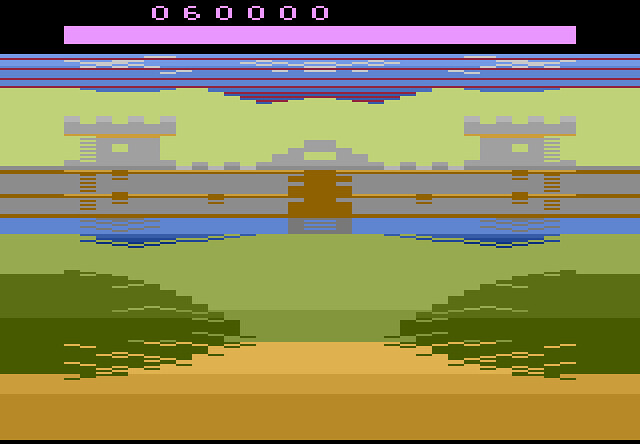The image appears to be a screenshot of a retro computer game with highly pixelated graphics. At the top of the screen, a score of 060000 is displayed in a lilac color within a black banner. Beneath this, a digital sky composed of blue and white pixelated rectangles, representing clouds, stretches across the background. A series of colored stripes create the landscape, starting from the bottom with layers of dark brown, light brown, various shades of green, blue, more light and dark brown stripes, and shades of grey. These stripes form a scenic view featuring what looks like a castle with a moat. The blue stripe depicts the moat surrounding the castle, while the shades of green represent the lawn and grassy areas. The brown lines suggest pathways or muddy areas, and the overall stripe pattern gives the impression of a castle nestled within a diverse terrain of water, grass, and sand.